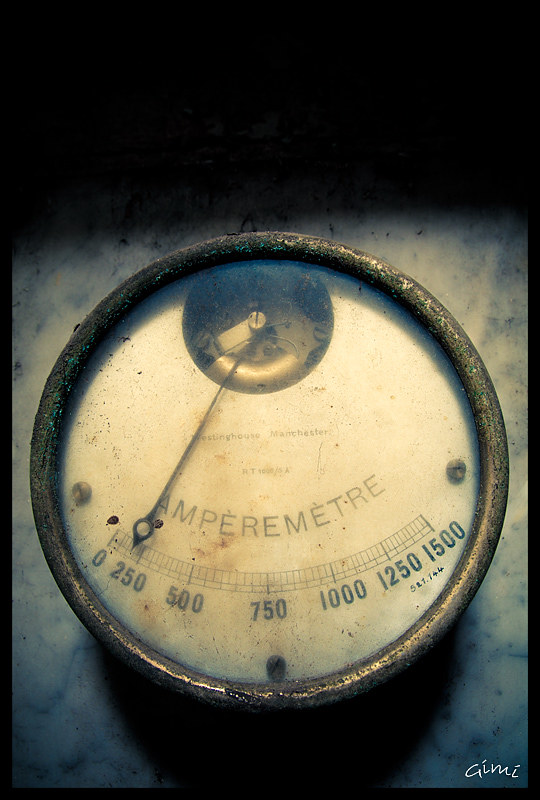Caption: An intricate close-up of a vintage temperature gauge, its exterior marked by the passage of time with a rusted silver casing. The gauge face, classic in white, displays a sequence of black numerical increments from 0 to 1500. Clearly designed for measuring extreme heat, its exact application remains a mystery. The French word "AMPEREMETRE" arcs across the dial, hinting at its foreign origin. A closer look reveals the finely crafted interior, where brass mechanical parts and even a small bell are visible through a purposely designed transparent section at the top. This antique piece, with its meticulous detailing and aged charm, speaks of a bygone era in engineering.